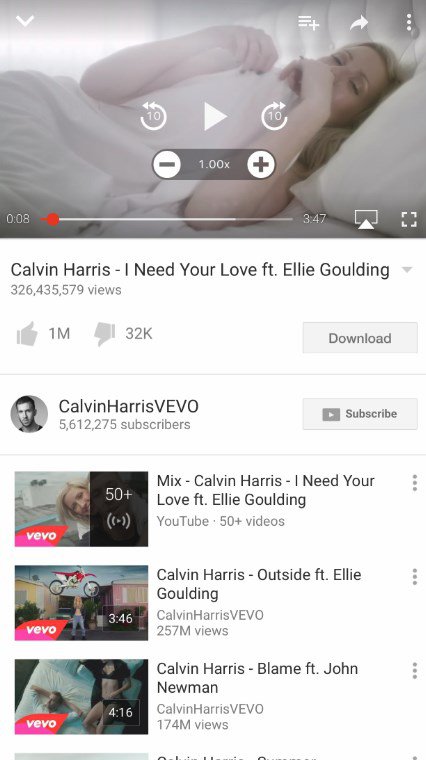Certainly! Here's a detailed and cleaned-up caption for the described image:

---

The image depicts an online interface, resembling a screenshot from a video streaming platform, possibly YouTube. The primary focus is on a rectangular landscape video at the top, featuring a woman lying down on a bed. She is positioned slightly diagonally, with her head to the right and her body oriented to the left. Her bare arms are bent at the elbows, with her hands near her face. To the right of her head is a pillow. The interface shows standard video controls in the center, including icons for rewinding 10 seconds and fast-forwarding 10 seconds. Below these controls, written in gray, is the playback speed option displayed as "1.00X," with buttons to increase or decrease the speed. A progress bar indicates that 8 seconds of the video have been watched, out of a total duration of 3 minutes and 47 seconds.

Directly beneath the progress bar is a gray text label stating "Calvin Harris - I Need Your Love ft. Ellie Goulding," identifying the video as a music video. Below this title, the view count is displayed as "326,435,579 views," indicating over 326 million views. Accompanying the view count are thumbs icons signifying likes and dislikes: the thumbs up shows "1M" (one million likes), and the thumbs down shows "32K" (32,000 dislikes). To the right is a download icon.

Further down is a channel information section showing a male icon and the text "Calvin Harris VEVO," with "5,612,275 subscribers" listed below the channel name. An adjacent rectangular button invites viewers to "Subscribe."

Underneath this main section, there are three horizontally stacked video suggestions, each with a thumbnail image on the left and title information on the right:
1. The first suggested video is "Mix - Calvin Harris - I Need Your Love featuring Ellie Goulding."
2. The second is "Calvin Harris - Outside ft. Ellie Goulding."
3. The third is "Calvin Harris - Blame ft. John Newman," noted with "174M views" for the bottom video.

All suggested videos feature the "VEVO" label on the left side of their thumbnails, each containing various images related to the respective music videos.

---